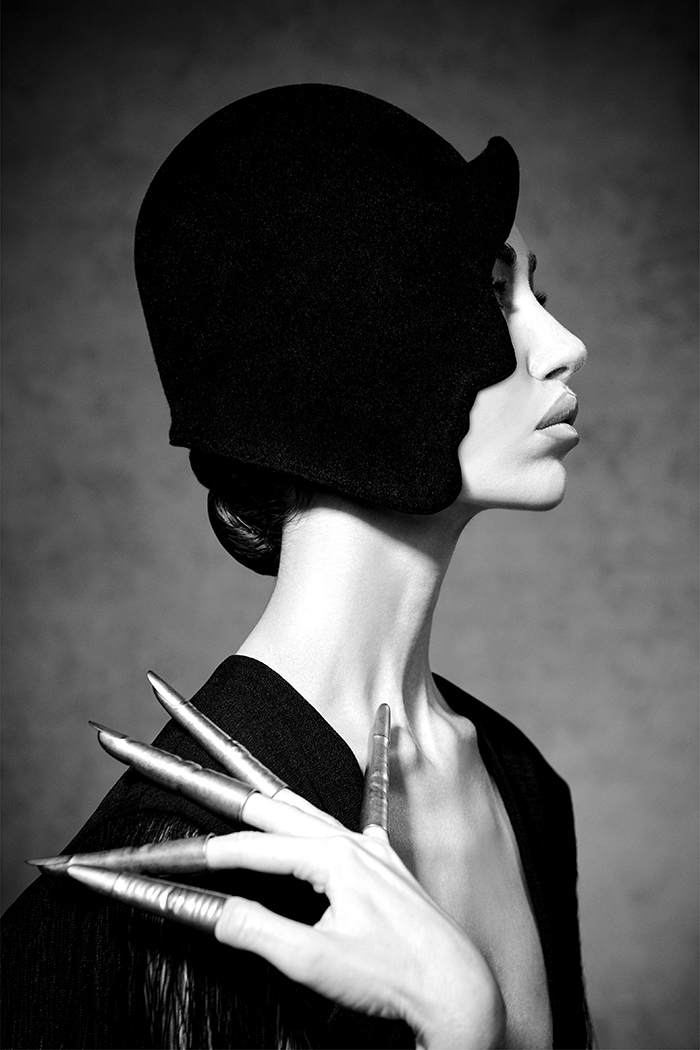In this black and white, vertically rectangular photograph, a slender woman of white ethnicity is captured from the shoulders up, standing in a dark gray backdrop. She faces to the right, showcasing a striking side profile with well-defined facial features—a prominent nose, full lips, and a rounded but sharply defined chin. Her makeup is subtle yet highlights her features, and her hair, styled into an abundant bun, is tucked away beneath a distinctive black hat. This hat fits snugly against her head and covers part of her forehead, extending down to her chin and adding an artistic touch with its human face-like shape, including a nose-like protrusion on the side. The woman is adorned in a black top, the exact style indeterminate, possibly a dress. Her left hand is elegantly placed on her shoulder, displaying extraordinarily long, light gray nail extensions or finger coverings that taper to metallic points, adding an avant-garde element to the image.